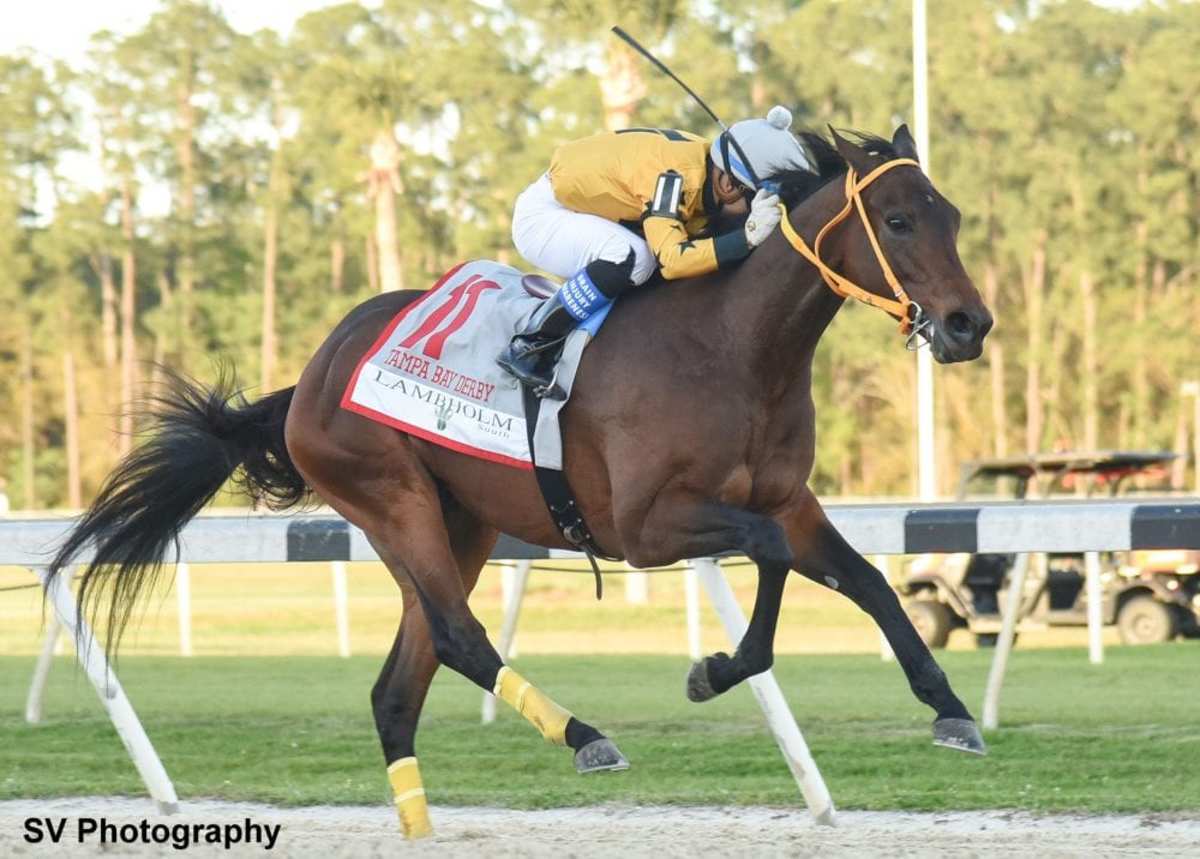This professional photograph captures a moment during the Tampa Bay Derby, featuring a sleek brown racehorse with distinctive black legs, tail, and mane. The horse is captured mid-gallop with three legs off the ground, illustrating its powerful stride. Adorned in a yellow bridle and yellow sleeves on its hind legs, the horse carries an intensely focused jockey. The jockey, wearing a yellow shirt, white pants, black boots, and a white helmet, is crouched low, his face buried in the horse's mane, possibly concentrating or indicating the high-speed intensity of the race. A whip is clenched in his hand, ready for use. The horse's saddle, an English style, bears the inscription "Tampa Bay Derby Lammheim South" on a gray and white blanket trimmed in red. The backdrop includes a white fence with black spots, a camouflage-patterned jeep, and blurred trees, all concurring the primary focus on the dynamic duo. The bottom left corner of the image is watermarked with "SV Photography," marking the artist's work.